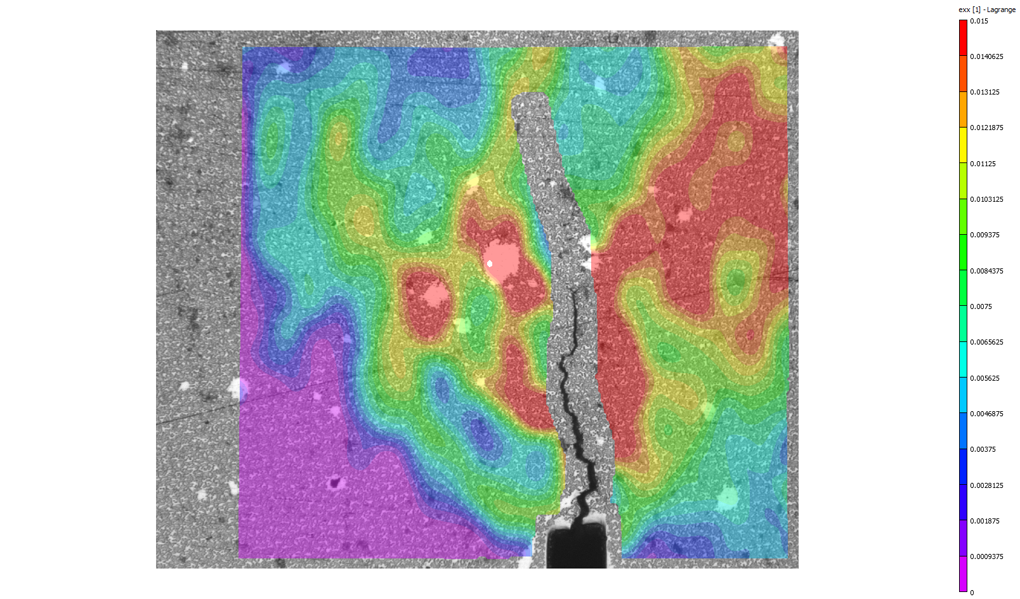This image appears to be a detailed heat map set against a gray, black, and white spot background. The central map section is a vibrant display of colors—ranging from deep purple and blue, through green and aqua, to intense yellow, orange, and red—indicating varying levels of intensity. The bottom left corner distinctly shows a fuchsia hue. Blue and aqua lines traverse the map, while a gray "river-like" band runs vertically through the middle, intersected by a prominent black line. This gray area also envelops other regions of color on the map. Within the map’s colors, the red, orange, and yellow tones dominate the right side, representing the highest intensity levels, whereas the cooler blues and purples are more prominent in the bottom left, top left, and bottom right sections. Adjacent to the right side of the main map, there's a boxed scale, likely indicating numerical values corresponding to the color intensities. Some white spots peek through the colored overlay, adding to the complex visual representation.